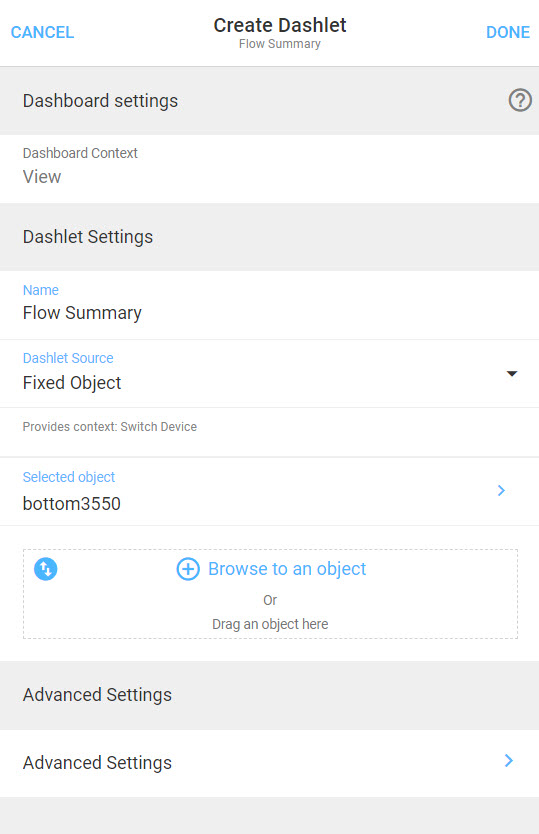This is a detailed screenshot from a phone displaying a user interface for creating a dashlet titled "Flow Summary." 

At the top-left corner, there is a "Cancel" option. The central header of the screen reads "Create Dashlet: Flow Summary." The background of the interface is white, while several boxes and elements are shaded in gray.

The first section is labeled "Dashboard Settings," which is shaded in gray. To the right of this label, there is a small circle with a question mark inside it, next to the text "Dashboard Context View." Below this, another gray-shaded section is titled "Dashlet Settings," followed by the heading "Flow Summary."

Next, there is a label "Dashlet Source" with a dropdown arrow next to the text "Fixed Object," indicating that a selection can be made from a list. Below "Fixed Object," the text "Provides Context Switch Device" is shown, followed by the label "Selected Object" with the value "Bottom 3550."

Further down the interface, there is a faint gray-outlined box. Inside this box, on the left side, there's a blue circle featuring an up and down arrow, along with a circle containing a plus sign. The adjacent text reads "Browse to an object or drag an object here."

Towards the bottom, there is a gray box labeled "Advanced Settings," followed by a white box with the same label, "Advanced Settings," which includes an arrow that suggests more information can be accessed via expansion.